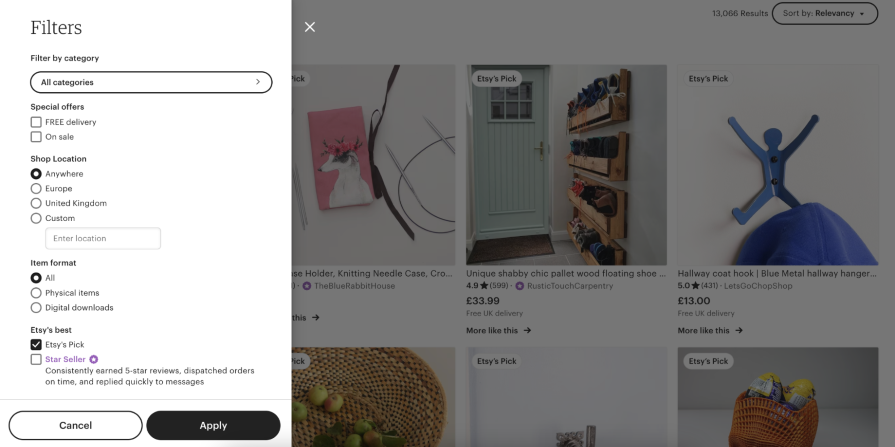The image depicts a detailed menu interface for filtering search results. 

At the top, the menu header reads "Filters," followed by a section titled "Filter by Category" with a text box that says "All categories." Below this, there are options for "Special Offers," each accompanied by a checkbox: "Free Delivery" and "On Sale."

Further down, there's a "Shop Location" section with options for "Anywhere," "Europe," "United Kingdom," or a custom location, prompting the user to set an interlocation. 

Next, the "Item Format" section presents three choices: "All," "Physical items," and "Digital downloads," each represented by circles suitable for selection. The "All" option is currently selected, marked by a black circle.

Additionally, the "Etsy's Best" section features two options, "Etsy's Pick" and "Star Seller." A description in purple text notes that these options include sellers who consistently earn five-star reviews, dispatch orders on time, and reply quickly to messages. The checkbox next to "Etsy's Pick" is selected and marked with a black checkmark.

At the bottom of the menu, there are two buttons: a white "Cancel" button on the left and a black "Apply" button on the right.